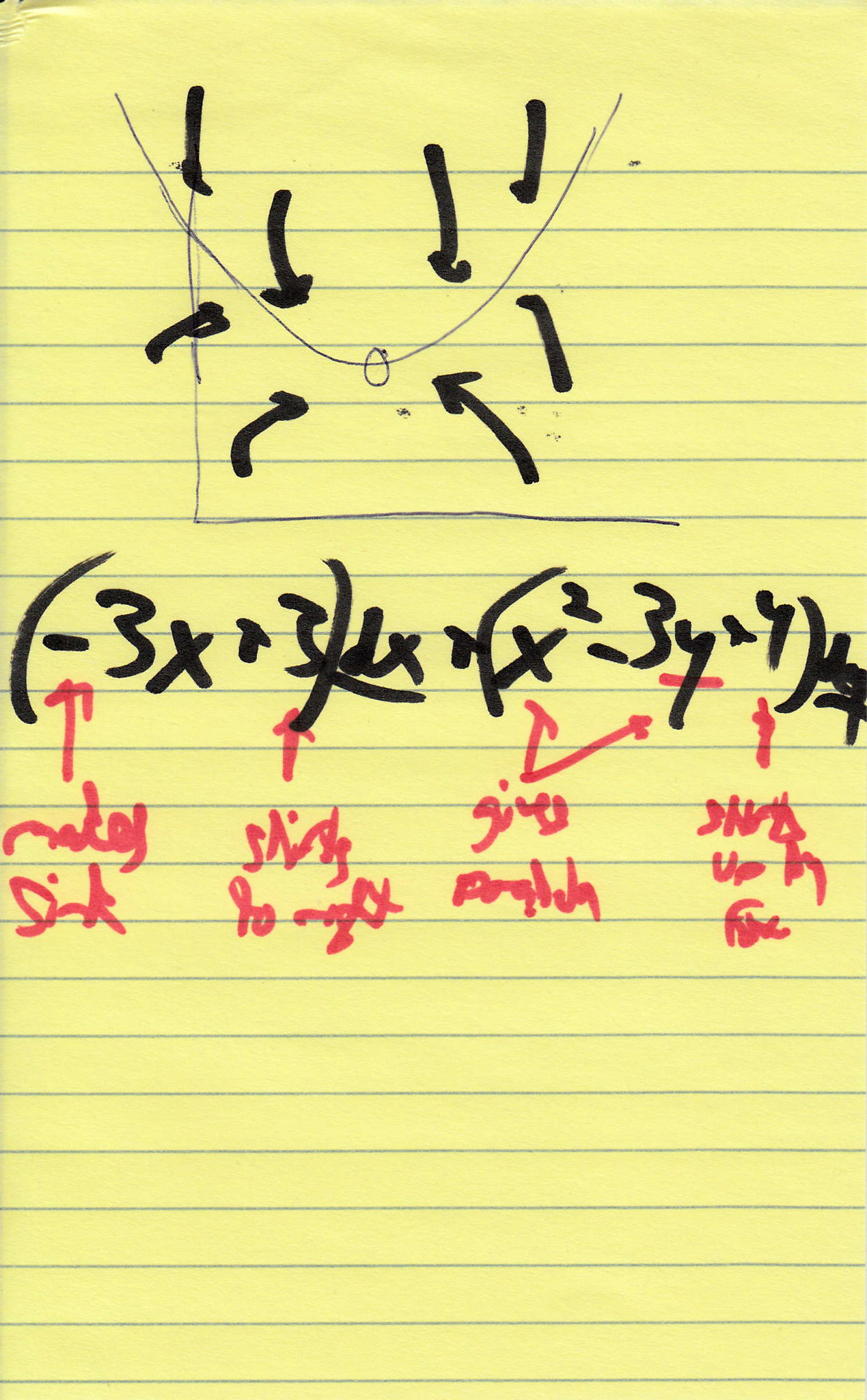This image features a piece of yellow notebook paper adorned with thin blue lines, showing a slight wrinkle in the top left corner. In the upper section of the page, there are ink-drawn markings: arrows pointing to a blue circle that has a blue line curving through it like a necklace. Centered on the page, written in black marker, is a combination of mathematical expressions that include negative 3 times what appears to be plus 3 DX, X squared, and other terms ending in minus 3, 4, plus 4. On the right side of this central content, an illegible scribble is present. Below these expressions, red ink inscriptions read "mates sinking" and possibly "sinks to right and gives…" with the final words remaining unreadable. Arrows in red ink connect these annotations to the central mathematical equations.